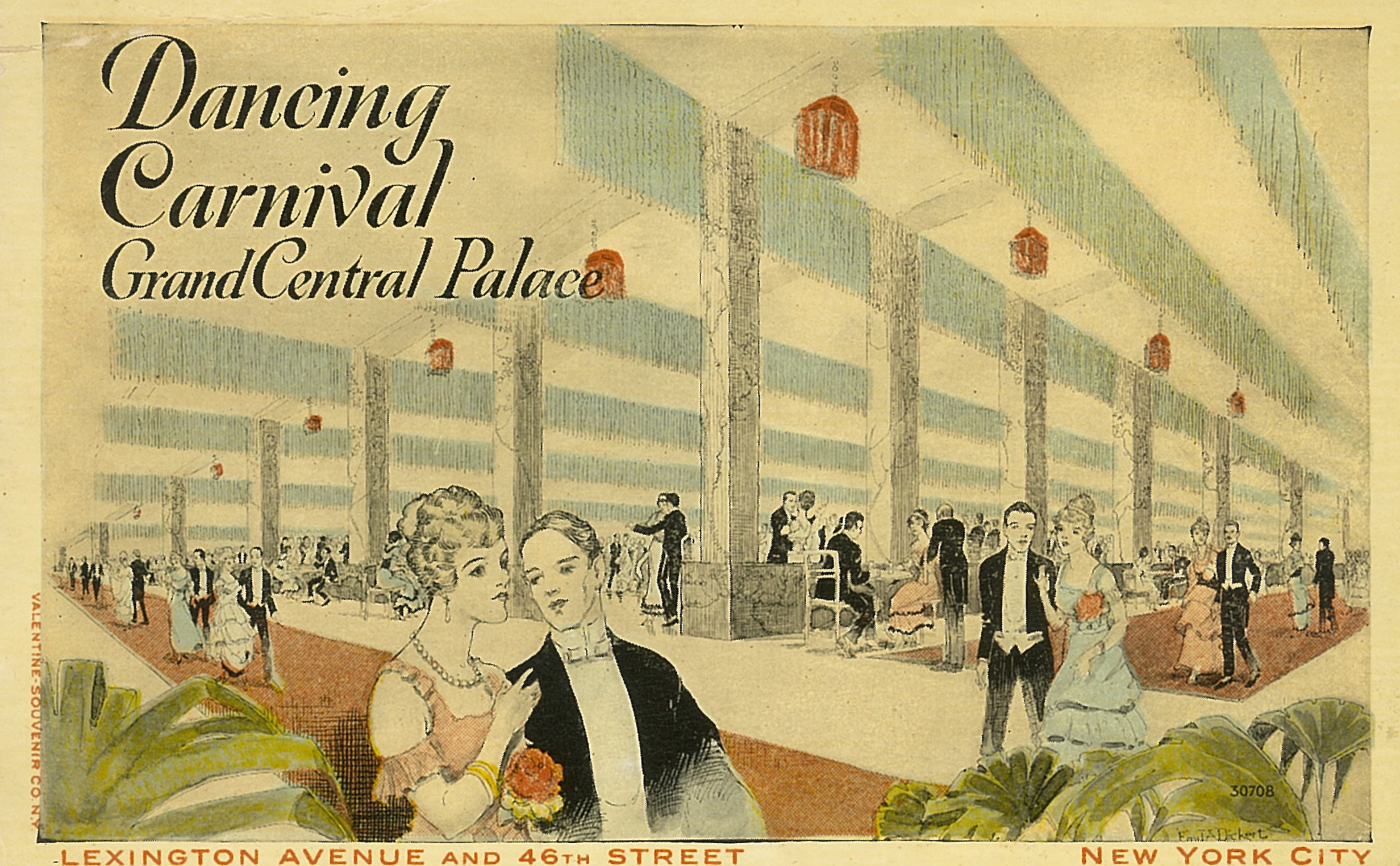In this illustration, the scene is set in the upper left corner with a prominent sign reading "Dancing Carnival Grand Central Palace" in green letters. The venue features an elegant green and white ceiling supported by a series of white columns. Adorning the ceiling are intricate brown lanterns that add a warm, inviting glow to the room. The ambiance is further enhanced by lush green plants strategically placed along the edges of the space. The flooring is a combination of white carpeting in the central area, surrounded by a polished brown wooden perimeter. The room is filled with well-dressed couples; the men are in immaculate black tuxedos paired with bow ties, while the women wear stunning long gowns in shades of blue, pink, and white. The overall atmosphere is one of sophistication and charm, further accentuated by the abundance of beautiful plants encircling the dance floor.